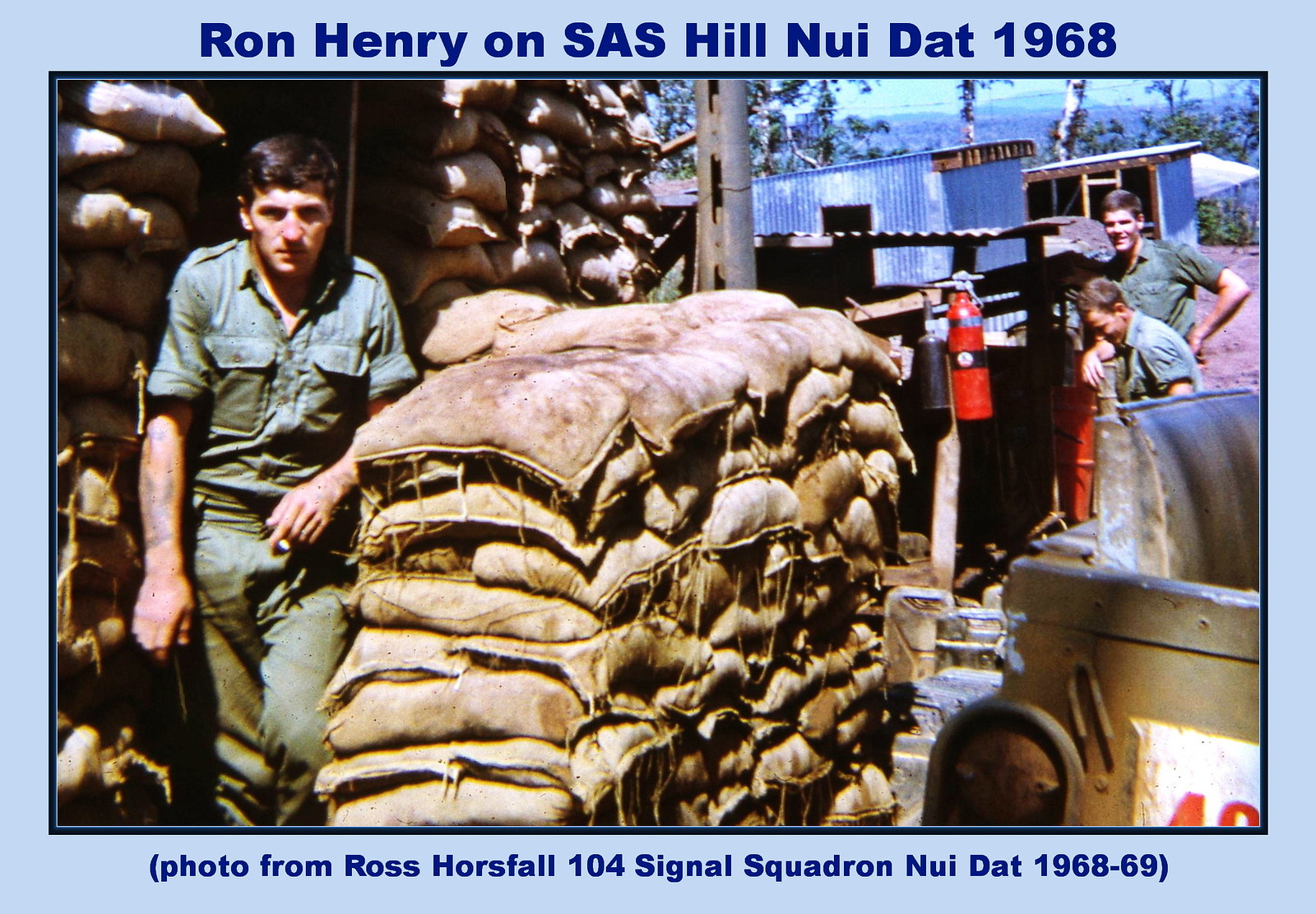The photograph shows an infantryman in a green military uniform, positioned behind a pile of sandbags on the left side. His brown hair and stern expression are visible as he looks towards the camera. In the background, two other soldiers, also dressed in green military attire, are seen near a couple of small huts, smiling and laughing. The scene appears to be set on a military base, possibly a Vietnamese base, with burlap bags piled high and fire extinguishers scattered around. The blue-bordered photo features text at the top reading "Ron Henry on S.A.S. Hill, Nui Dat, 1968," and at the bottom, it notes, "Photo from Ross Horsfall, 104 Signal Squadron, Nui Dat, 1968-69." The sky is slightly visible in the distant background, adding depth to the outdoor setting.